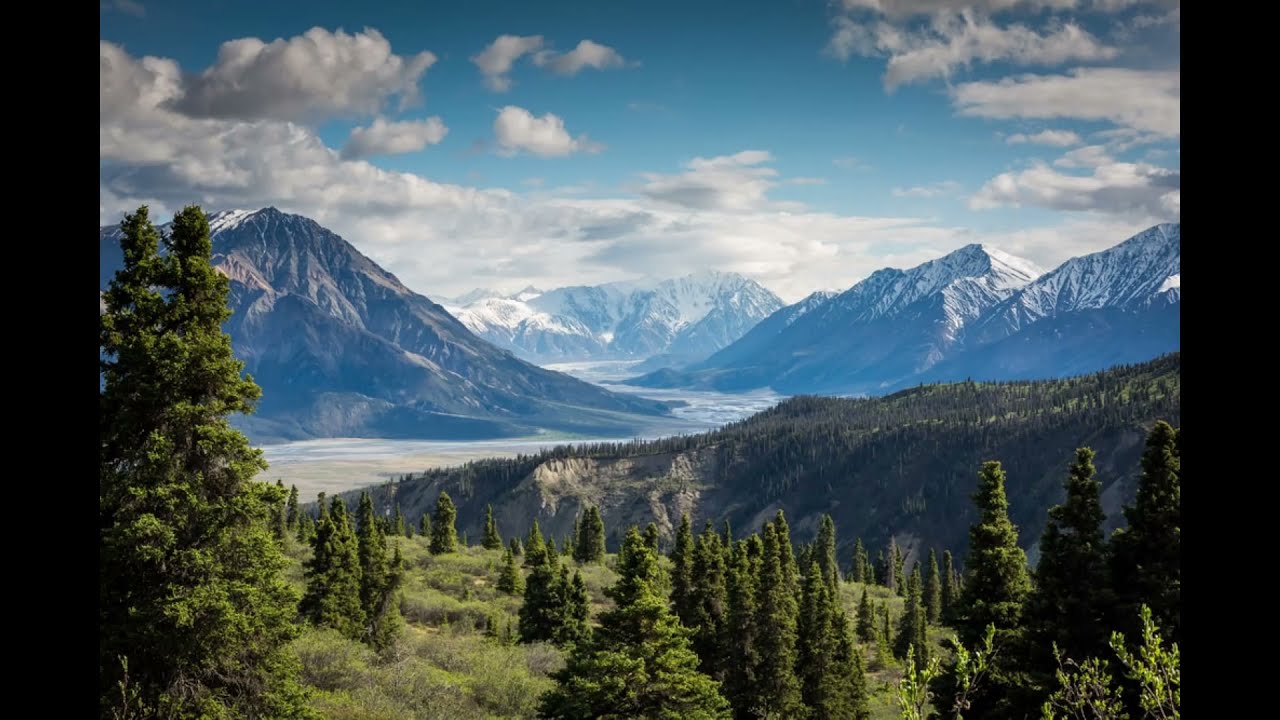The image captures a stunning and seemingly surreal landscape scene, encompassing a variety of natural elements in striking detail. In the foreground, scattered evergreen pine trees rise amidst thick green vegetation and unkempt grass. These trees are denser on the left side, creating a natural frame for the scene. Beyond this, the terrain falls off sharply, resembling a steep cliff. From here, a more rugged, rocky mountain ascends almost vertically with a light brown hue and sporadic tree coverage.

The midsection of the image features a winding river that originates from the left, snakes through a lush valley, and flows towards the center before disappearing into the backdrop of the mountains. The water's path contributes to the dynamic composition of the picture, infusing it with a sense of motion.

In the background, imposing snow-capped mountains rise majestically, their peaks solid rock and glistening with snow that extends halfway down their slopes, transitioning into grey and black hues lower down. The farthest peaks are heavily snow-laden, contrasting starkly with the rugged slopes below.

The sky above is a patchwork of light and dark blue with clouds scattered throughout. Some clouds are thick and grey, hinting at rain, particularly on the left side, while others are white and fluffy, adding texture to the blue expanse.

Overall, the scene is a blend of rich natural beauty and an almost uncanny, hyper-realistic clarity that makes it feel like a 3D rendering despite its seemingly authentic features.